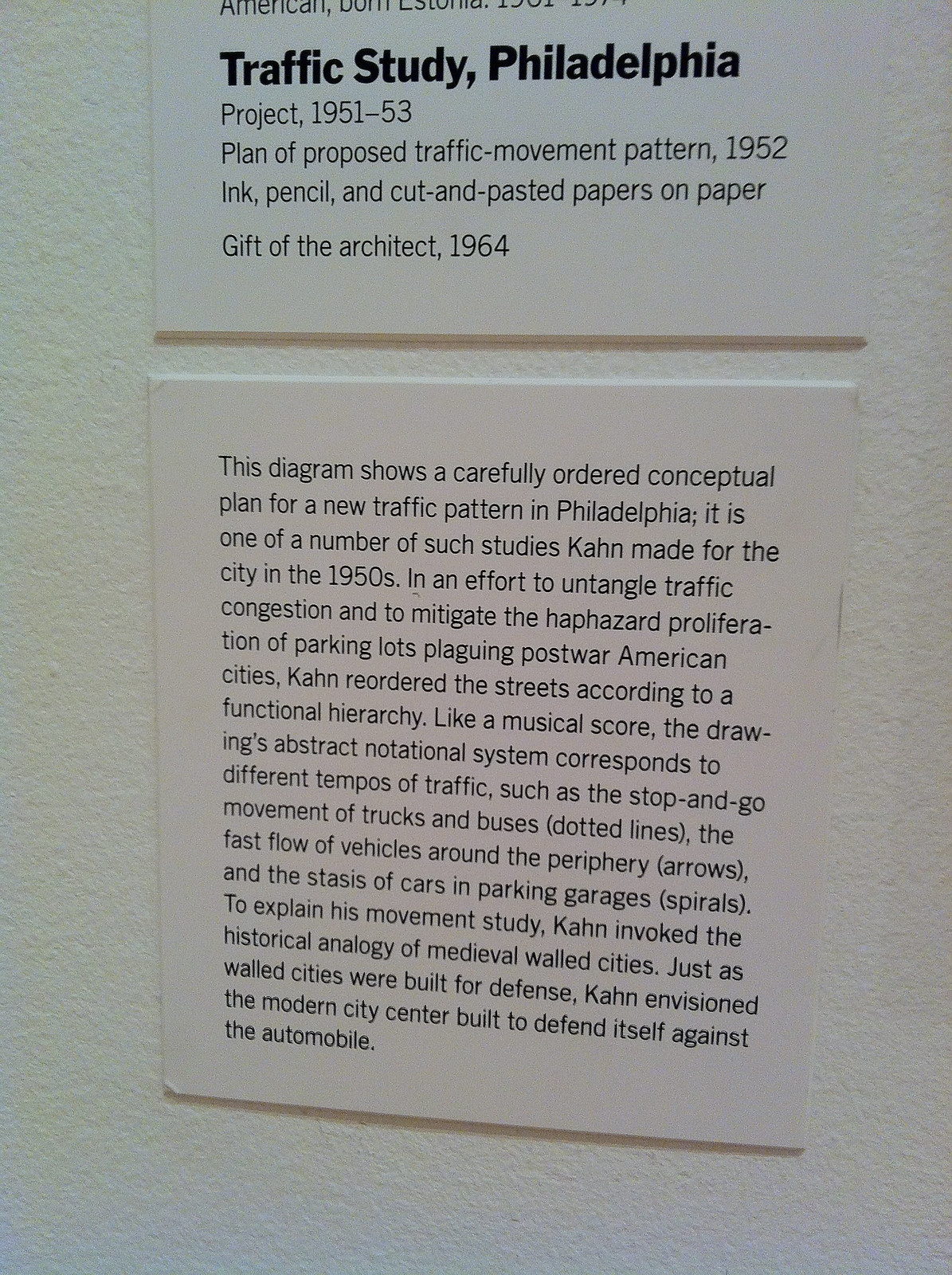The photograph showcases two descriptive white cardstock signs with embossed black text mounted on a textured, off-white brick wall. The first, a horizontal piece, reads: "Traffic Study, Philadelphia, Project 1951-53, Plan of Proposed Traffic Movement Pattern, 1952, Ink, Pencil, and Cut and Pasted Papers on Paper, Gift of the Architect, 1964." This indicates it's a museum exhibit featuring a historical traffic study project. Below it, a vertical sign elaborates on the project's purpose, explaining that the diagram presents a thoughtfully ordered conceptual plan for a new traffic pattern in Philadelphia. Created by Kahn in the 1950s, it aimed to alleviate traffic congestion and manage the spread of parking lots in post-war American cities by reorganizing the city's streets into a functional hierarchy. The diagram uses a symbolic notational system akin to a musical score, representing various traffic tempos—stop-and-go (dotted lines), fast-moving periphery traffic (arrows), and static parking (spirals). Kahn compared this modern traffic strategy to medieval walled cities designed for protection, suggesting the modern urban center should defend itself against automobile chaos.